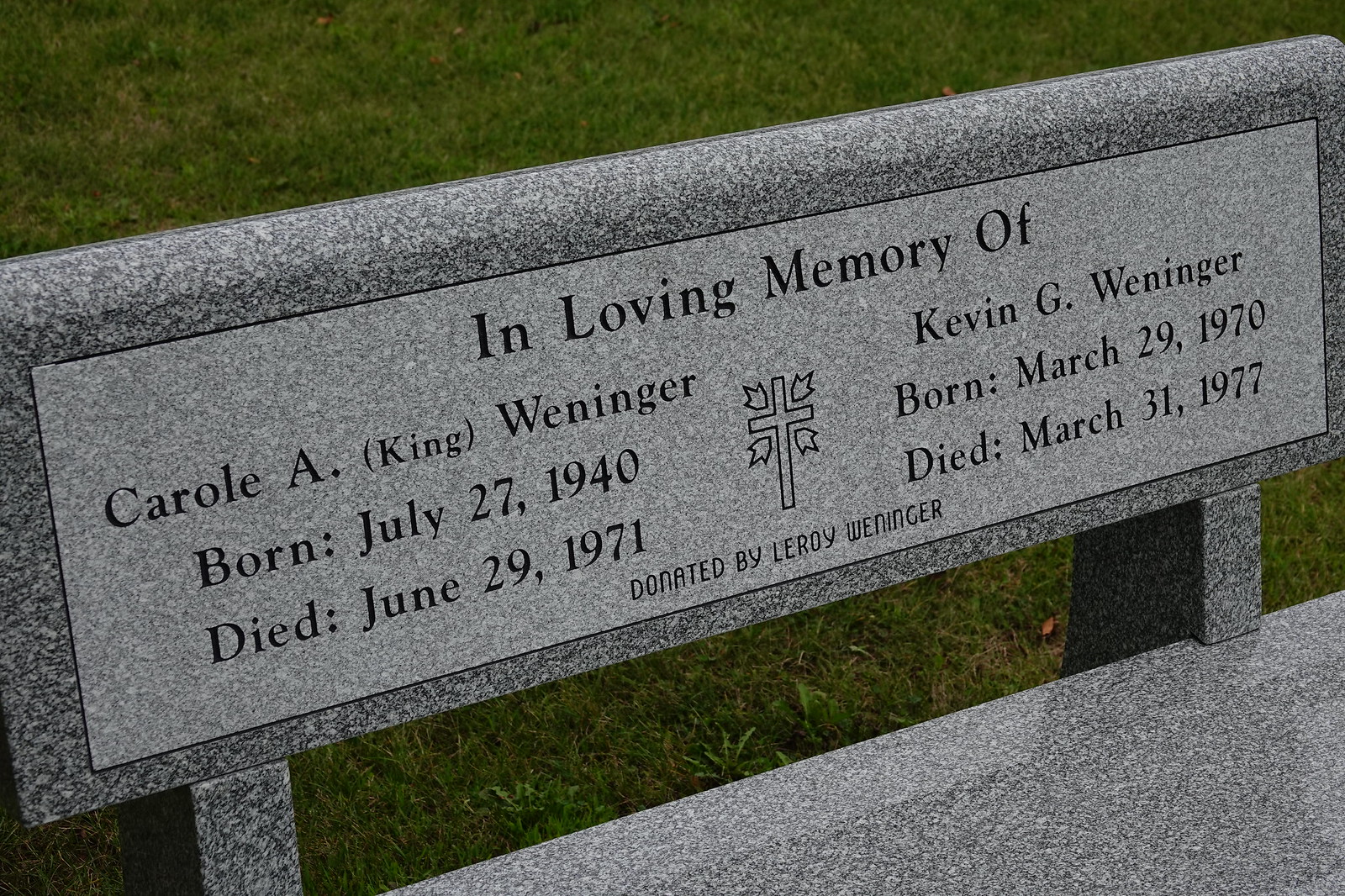The image depicts a stone bench, likely situated in a cemetery or park, surrounded by green grass. The bench, made of dark gray stone with a lighter inset stone, bears a detailed inscription in black letters. The top of the inscription reads "In loving memory of." Below, on the left, it commemorates Carol A. (King) Wenninger, born July 27, 1940, and died June 29, 1971. On the right side, it honors Kevin G. Wenninger, born March 29, 1970, and died March 31, 1977. A Christian cross is also etched into the stone. At the bottom of the inscription, it is noted that the bench was "Donated by Leroy Wenninger." The image was taken during the daytime, providing a clear view of the green grassy background surrounding the bench.